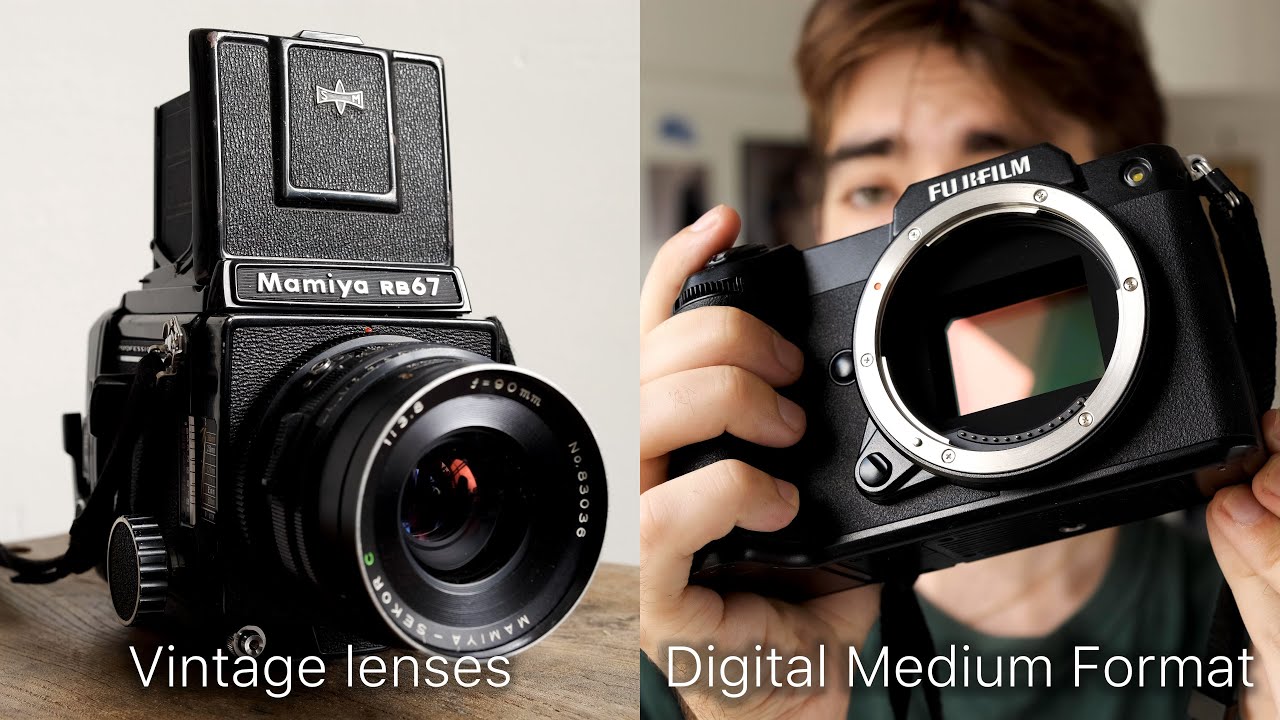This image presents a side-by-side comparison of two cameras. The left photo features a vintage Mamiya RB67 camera, identifiable by its front-facing black body and protruding lens that bears small, indistinct white text. A knob on the viewer's left and a black cord are also visible. This image, set against a white wall and showing the camera on a table, is labeled "Vintage Lenses" in white text at the bottom. The right photo shows a person, mostly obscured except for a green t-shirt, holding a modern Fujifilm camera with a large, flat lens that reflects a rectangular shape. The camera, also black, includes white text at the top spelling "Fujifilm" and a black cord hanging down. The slightly out-of-focus background reveals part of the house but lacks discernible details. This photo is labeled "Digital Medium Format" in white text at the bottom.